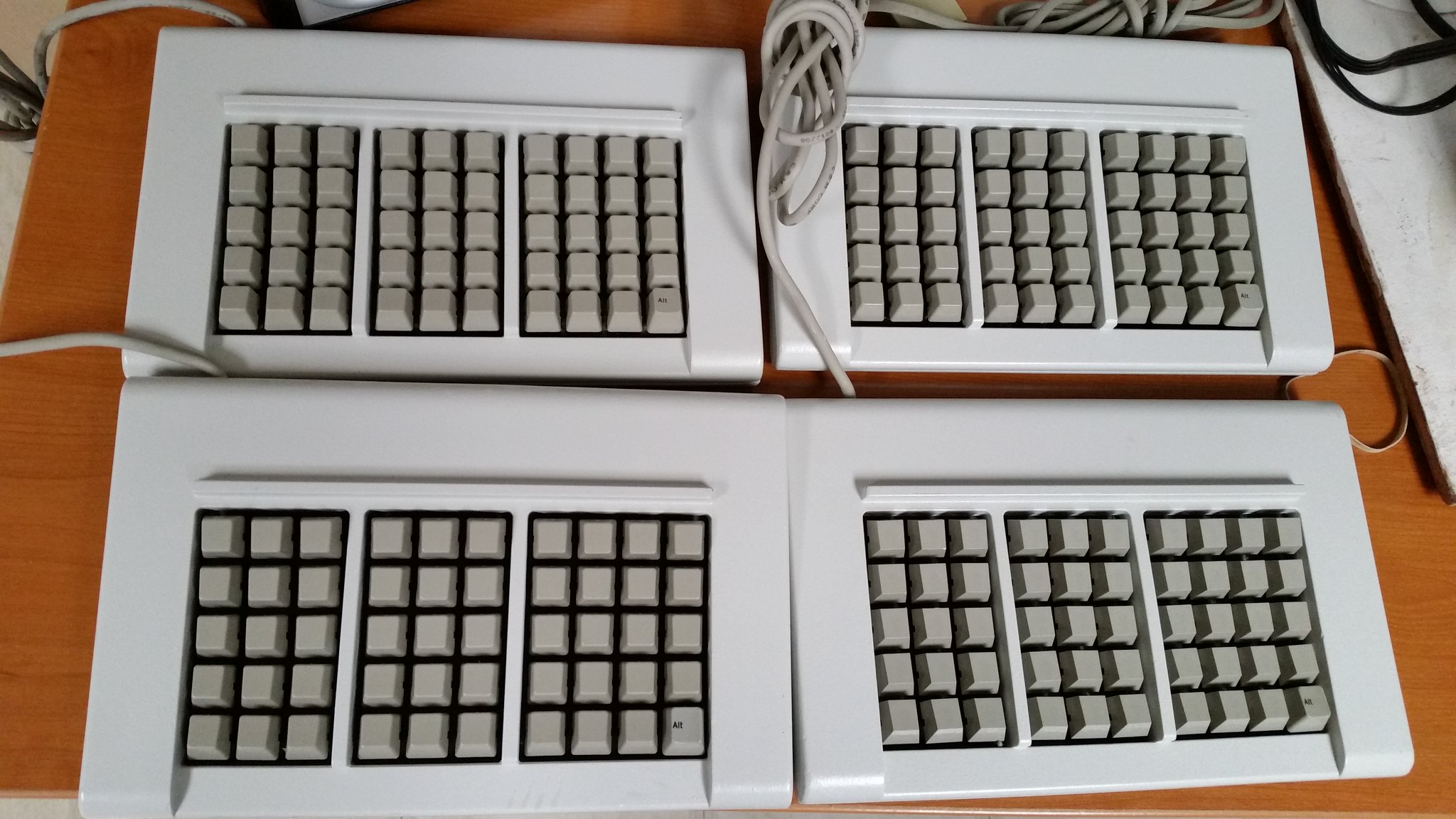The image showcases a close-up of four distinct, early prototype keyboards, positioned on a reddish-brown wooden table. Each keyboard features a different array and configuration of keys with no alphanumeric characters, except for a single 'Alt' key on the far right. The keyboards, made from a taupe white plastic, vary in layout: two of them have a 3x5 arrangement, while another follows a 5x4 pattern, and the fourth is slightly different. The keys themselves are a darker gray compared to the lighter gray of the keyboard bodies. Grey wiring extends from each keyboard, with a coil of it placed between the top two keyboards. The photograph is simply composed with no additional text or signatures.